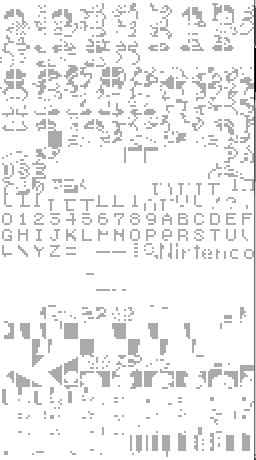This image presents a highly unique and abstract composition. Central to the scene is a stark white page, with a prominent, long black line running along one side. The background is adorned with various abstract, gray spirally shapes, flanking both the top and bottom of the image. Interspersed among these spirals are gray boxes and shapes that bear a passing resemblance to elements such as bunny ears and rudimentary robot-like figures.

In the center of the image, a string of letters and numbers appears in a bold, blocky old-school computer font. The text reads "n-i-r-t-e-n-c-o netaiko." Below this text, additional graphics emerge, growing more abstract and less definable as they descend. The graphics at the bottom lack the representational qualities of the upper shapes, though one might tenuously identify a figure resembling a dinosaur, marked subtly by features that could be interpreted as a smiling eye and mouth.

The upper graphics seem to intentionally blend elements of robots, people, and possibly bunnies, creating a curious amalgamation of forms. The purpose and meaning of the bottom graphics remain ambiguous and harder to delineate. Despite the abstract nature of the image, this mixture of recognizable and enigmatic shapes invites a deeper contemplation of its artistic intention.